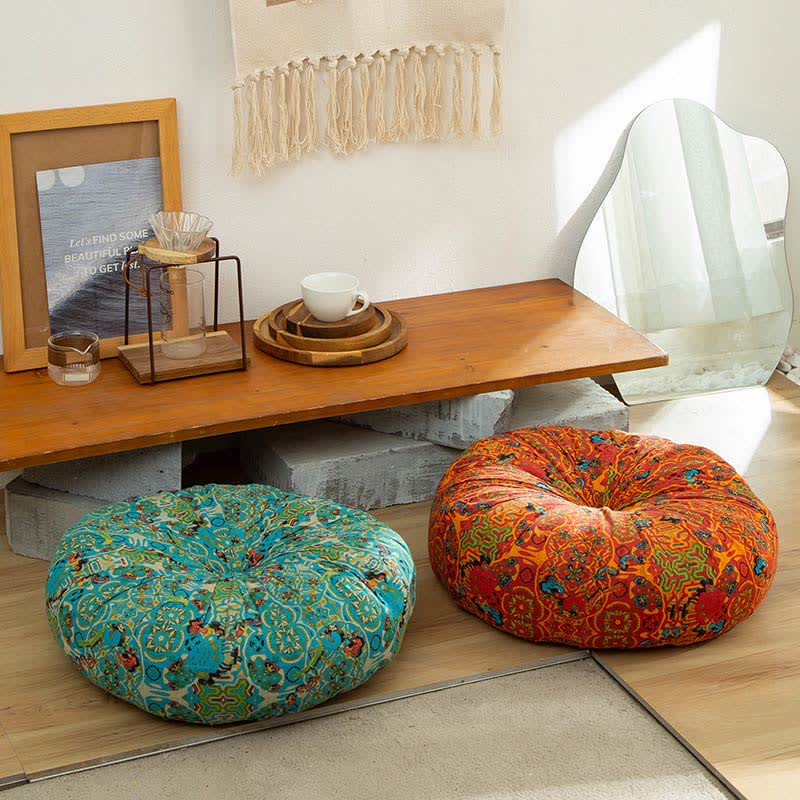The photograph captures a serene interior scene, likely a living room, with a meditative, Asian-inspired ambiance. Central to the composition are two roundish beanbag chairs with button dimples resembling cooked bagels; one features a turquoise blue pattern interwoven with hues of light green, white, and a hint of red, while the other displays a predominantly red and orange motif with intricate mandala-esque designs. Positioned in front of these chairs is a unique, low wooden table with no visible legs, instead supported by stacked white concrete blocks forming a geometric base.

On the table lies a series of three nested, natural wooden trays, topped with a simple white teacup. Nearby, a decorative piece consisting of bracketed metal loops and a glass jar sits on a wooden disc, possibly serving as a candle holder. The table also supports a minimalistic wooden photo frame displaying a black-and-white image of a breaking wave, partially obscured by the décor, with an inscription encouraging exploration: "Let's find some beautiful places to get lost."

The wall behind the table features a beige cotton tapestry with tassels, adding a soft, artistic touch to the space. Resting against the wall in the right-hand corner is an amoeba-shaped mirror with a straight bottom edge, enhancing the room's eclectic feel. The environment is bathed in bright, natural sunlight, illuminating both the area with wooden plank flooring and the unfinished concrete surface, creating a harmonious blend of textures.